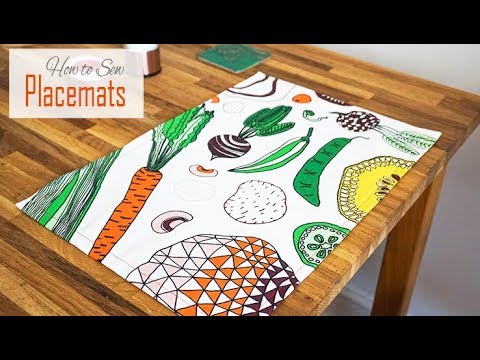Against a black background, the image prominently features a dark or medium green wooden table. Positioned on the table is a predominantly white, hand-drawn, artistic placemat, meticulously stitched along the edges. The design showcases an array of colorful vegetables, including an orange carrot, sliced mushrooms, peas, a pepper, lime and lemon slices, a radish or turnip, and possibly a cucumber and corn or melon. Some elements are left uncolored, adding a modern minimalist charm. In the upper left corner of the image, a rectangle contains text that reads "how to sew placemats," suggesting the image is part of a tutorial or advertisement. Behind the placemat, there is a green coaster and a metallic object, possibly a candle, adding depth to the scene.